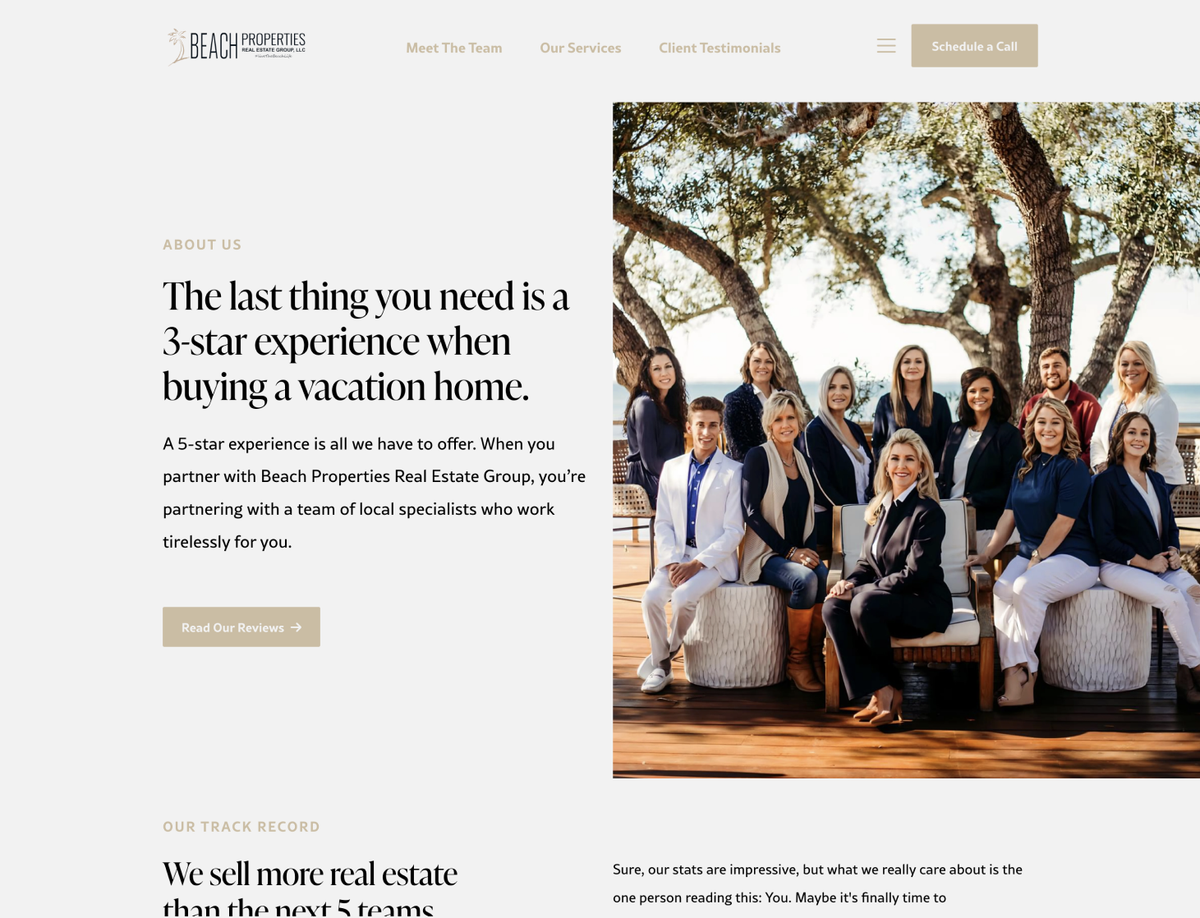A detailed description of a web page showcasing Beach Properties Real Estate Group. At the top, we find a brown graphic of a palm tree. The website's title, "Beach Properties," is prominently displayed in black font. The navigation bar features tabs in a tan color labeled "Meet the Team," "Our Services," and "Client Testimonials." To the right of these tabs are three horizontal lines, indicating a menu, and a "Schedule a Call" button in the matching tan hue.

Just below, a brown header reads, "About Us," followed by a slogan in black text: "The last thing you need is a three-star experience when buying a home. A five-star experience is all we have to offer when you partner with Beach Properties Real Estate Group. You are partnering with a team of local specialists who work tirelessly for you." 

Under this, a brown button prompts visitors to "Read Our Reviews." To the right of the text, an image features a group of professional individuals, positioned in front of an oak tree. The group consists of several women and two gentlemen, all dressed in business casual attire. Some members of the group are standing, while others are seated, and they are all smiling warmly at the camera.